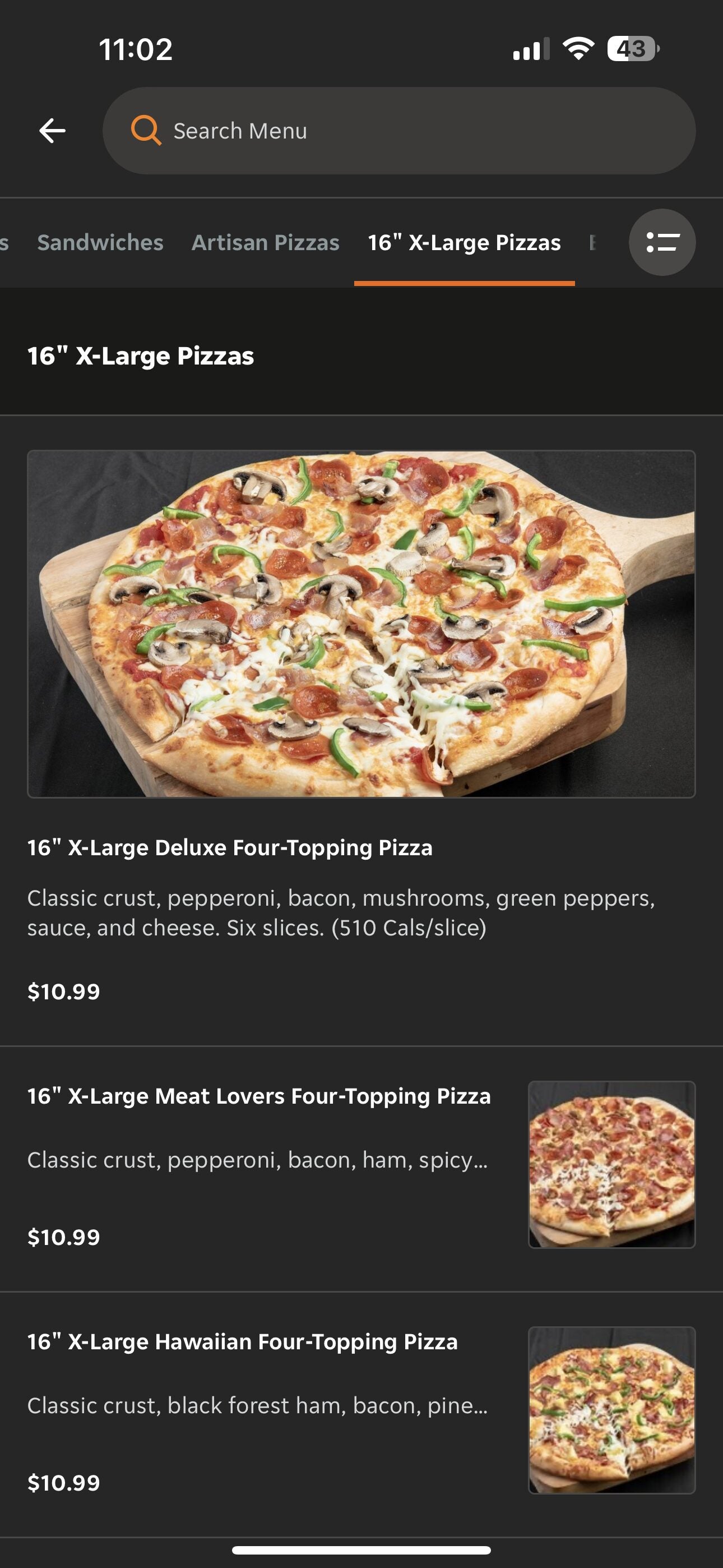This screenshot, taken at 11:02 with Wi-Fi enabled and the phone displaying a 43% battery level, features a searchable menu interface. At the top of the screen is a search bar reading, "Search Menu." Below the search bar, different menu categories are listed, including "Sandwiches" and "Artisan Pizza." Highlighted in this list is the "16-inch Extra Large Pizza" category.

The image prominently showcases a 16-inch extra-large pizza resting on a wooden paddle, typically used for handling the pizza in and out of the oven. The pizza is cut into six slices and is topped with pepperoni, green peppers, onions, and likely mushrooms. Below this image, it states "16-inch Extra Large Deluxe Four-Topping Pizza," detailing the ingredients as a classic crust base with pepperoni, bacon, mushrooms, green peppers, sauce, and cheese. Each slice contains 510 calories, and the pizza is priced at $10.99.

Beneath this section, the menu lists another option: a "16-inch Extra Large Meat Lovers Four Topping" pizza with a classic crust, including pepperoni, bacon, ham, and another ingredient that is partially obscured, priced similarly at $10.99.